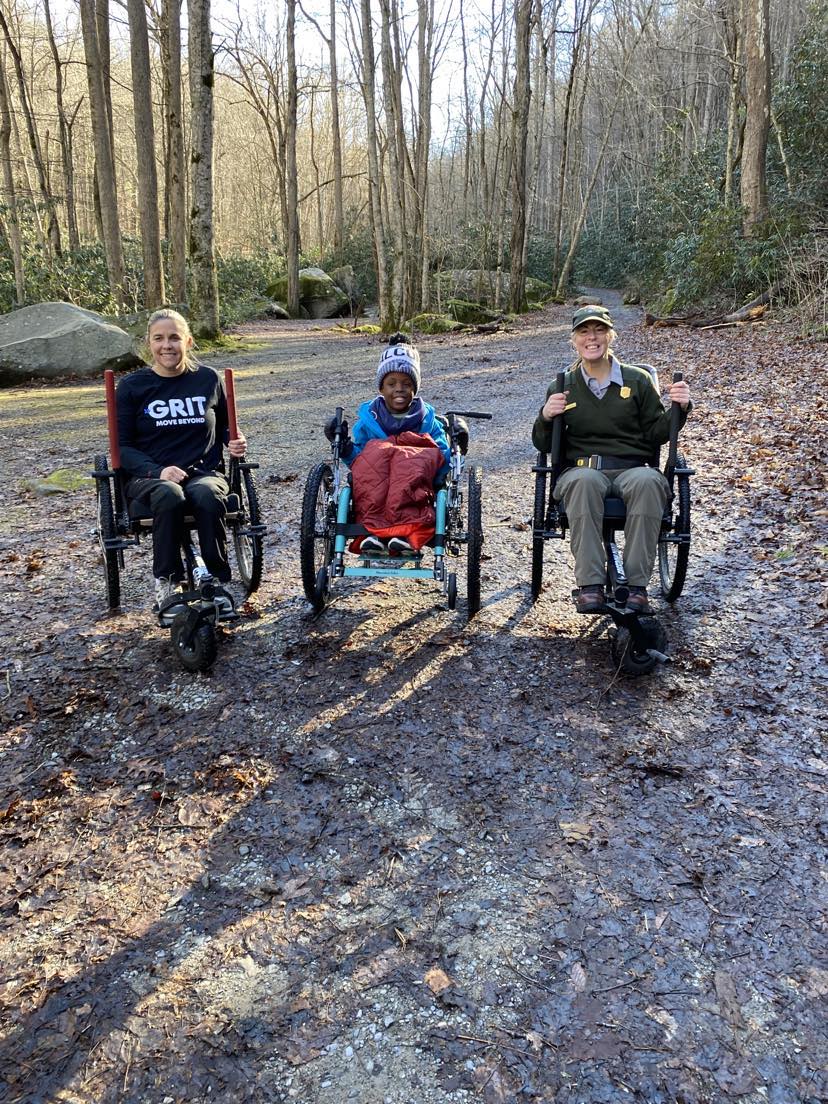The image depicts three individuals in wheelchairs situated outdoors in what appears to be an autumn or early winter setting. The ground is covered with dead, wet leaves, and the background reveals large, leafless trees, suggesting a forested area. The woman on the left, a white female with brown hair, is seated in a black wheelchair with red handles and a front wheel. She wears a long-sleeved blue sweatshirt with the word "GRIT" emblazoned in white text. The individual in the middle, a young black boy, is dressed in a blue jacket and a blue beanie, and has a blanket draped over his lap. On the right is another white female, dressed entirely in green with a matching sweatshirt, pants, and baseball cap. The scene is illuminated by daylight, and the group appears content and happy as if they have just enjoyed hiking or spending time in nature.